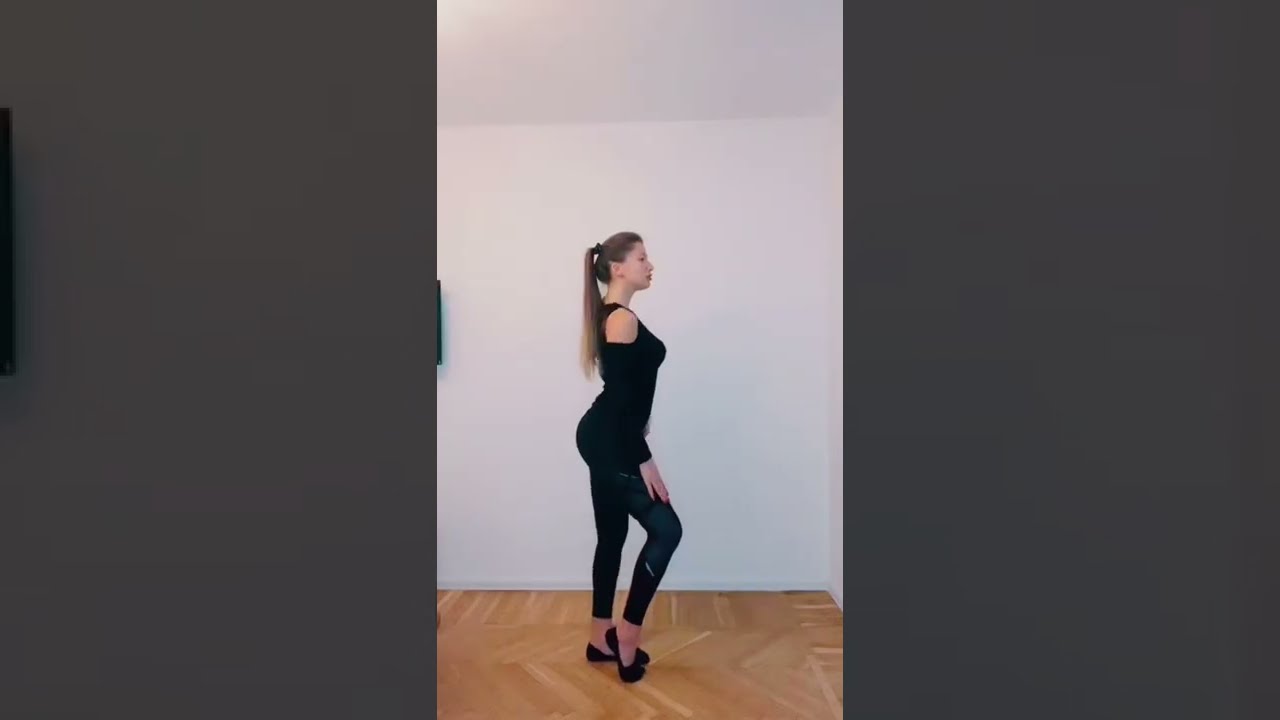In this image, captured within a dance studio, a young Caucasian woman in her 20s is poised for a dance routine. The setting features a clean, light brown bamboo hardwood floor and plain white walls, creating a minimalist backdrop. The studio is flanked by dark gray vertical panels on the left and right sides, centering the focus on the dancer. She is dressed in a tight black bodysuit with open shoulders, paired with black ballet slippers and arm warmers. Her long blonde hair is tied back in a ponytail. She stands with impeccable posture, her back arched straight and her chin slightly raised, as if studying her reflection in an unseen mirror. Facing the right side of the image, she has her right leg bent at the knee with her toes touching the floor and her right hand resting gently on her thigh. Her left leg remains straight, grounding her stance. The composition and her serene expression with closed eyes convey a moment of contemplation and grace, possibly a pause before launching into her dance routine. The overall impression is of a dancer deeply engrossed in her practice, in a moment of calm and focus.